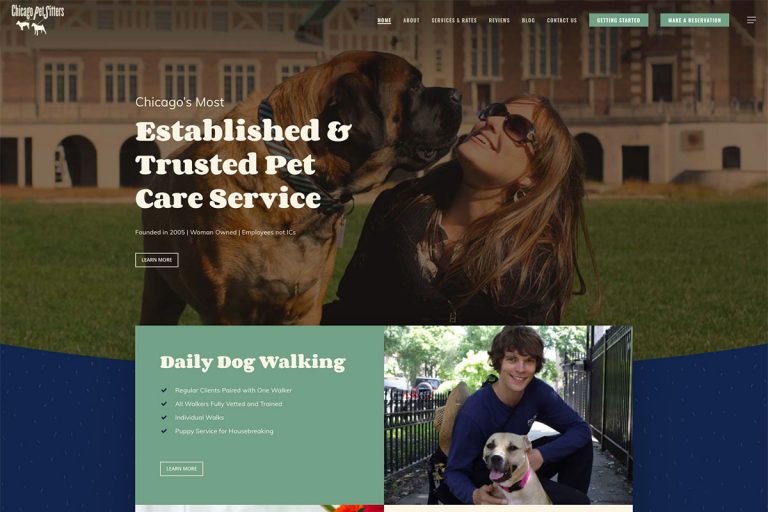The image showcases the website of "Chicago Death Citers," a well-established and trusted pet care service founded in 2005. The website navigation panel is visible on the right, featuring links such as Home, About, Services and Rates, Reviews, Blog, Contact Us, Getting Started, and Make a Reservation. The caption highlights that the business is woman-owned and employs staff rather than independent contractors (ICs). 

Key features mentioned include daily dog walking, assigning regular clients' pets to one dedicated walker, comprehensive vetting of all walkers, individualized logs, and specialized puppy services for house training.